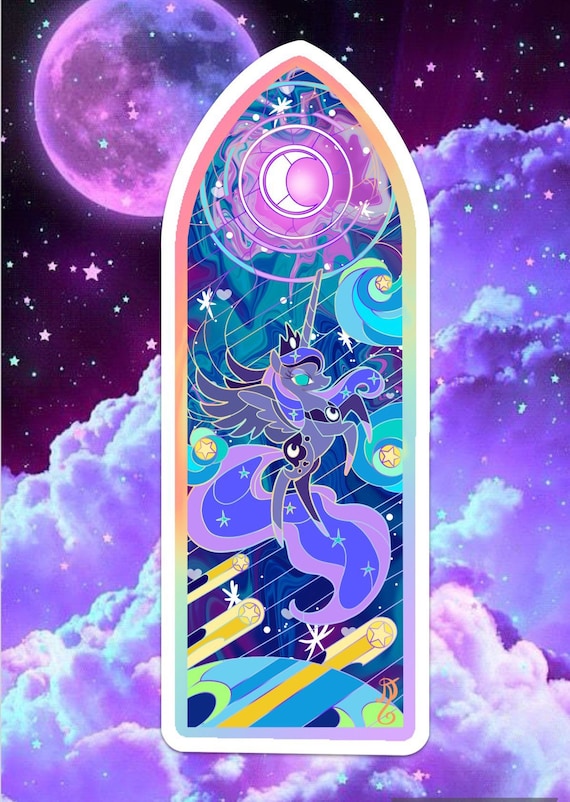This image is a vibrant computer graphic reminiscent of a stained glass design. At the forefront is a whimsical depiction of a small, baby purple unicorn with an oversized horn, large wings, and a big fluffy tail, resembling a majestic pegasus. The unicorn floats above a scene featuring geometric and cubist influences, composed of various vivid shapes in a color palette dominated by purples, blues, greens, pinks, and yellows.

In the background, a dreamlike sky is painted with pixelated clouds and a crescent moon that casts a mysterious purple haze, while star-shaped figures dot the scene. Additionally, a full moon joins the ethereal backdrop but isn't particularly bright. The stars look more like starfish than the typical star dots seen in night sky photographs, adding to the surreal atmosphere. Comets streak across the sky with yellow lines reminiscent of shooting stars. The lower part of the image includes an outline of the Earth, linking the celestial theme back to our world. The overall design creates a sense of a mystical, otherworldly night sky with a whimsical, fantastical centerpiece.